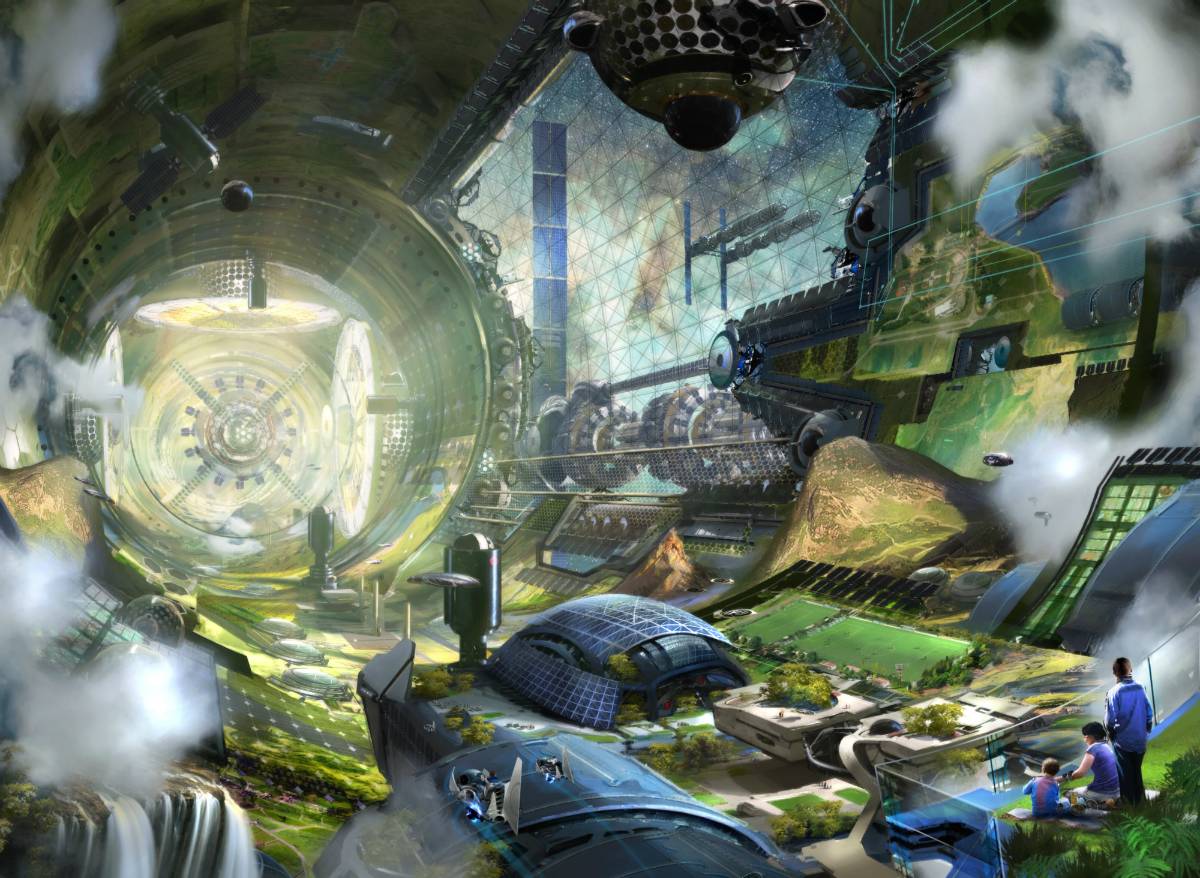The image portrays a vivid and expansive futuristic scene, likely a highly detailed digital artwork or AI rendering, reminiscent of spaces described in the Gundam series. The setting appears to be the interior of a colossal cylindrical structure, with the ground curving up along the walls. Within this gigantic tube, the environment blends natural elements and advanced technology. The bottom area features lush green fields and a central headquarters-like building, partially surrounded by metal frameworks and random bolts. A lucite or clear, see-through barrier separates the lush indoor habitat from three figures in the bottom right corner: a family comprising a seated mother and son, and a standing father. Overhead, the structure is dominated by large, churning gears and other metallic mechanisms, partially encased in glass through which the galaxy is visible. Additional details include cascading water, evoking a waterfall, and an intricate blue dome-style building with plant life sprouting from it. The cavernous space, filled with propeller-like elements and framed by clouds or smoke, exudes an almost museum-like, echoey ambiance, providing a stark juxtaposition of untouched nature and stark industrial design.